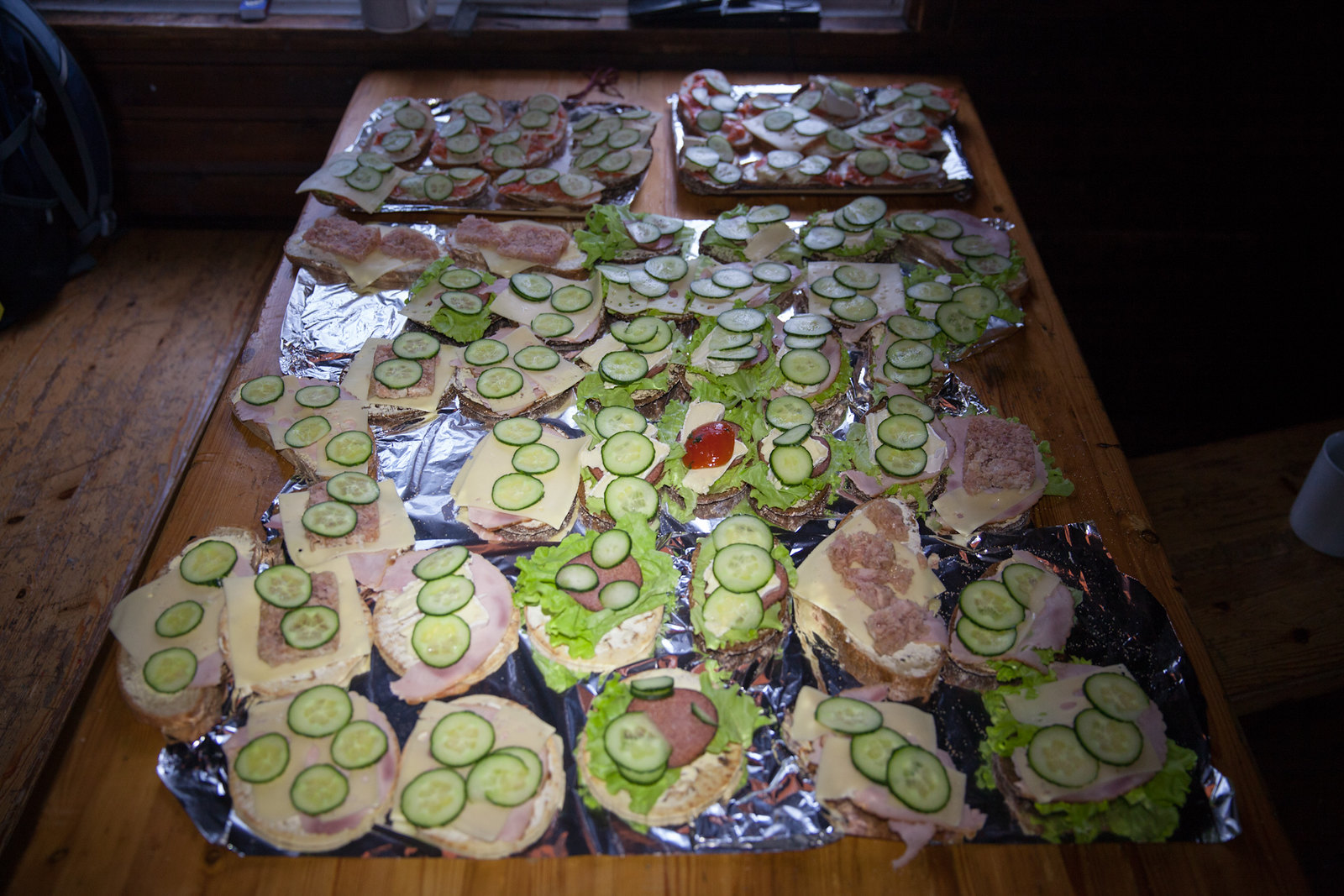The image depicts a dark indoor setting with a wooden rectangular table, likely situated in a restaurant, illuminated by some moonlight coming through a window in the background. The table, encompassing nearly the entire frame, is laden with numerous open-faced sandwiches arranged on aluminum foil. Each sandwich seems to be based on a slice of bread or possibly a bagel, topped with a variety of meats including ham, salami, and bacon. Many also feature slices of cheese, leafy lettuce, and prominently, cucumber slices. One sandwich has a notable addition of something red, potentially a tomato. The wooden floor beneath the table is visible, adding to the rustic atmosphere. The sandwiches are organized on trays that cover almost the entire surface of the table, making it appear ready for a large gathering or celebration.